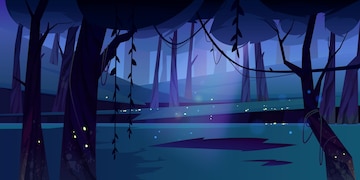The image is a tiny horizontal digital photo that appears to be taken with a phone camera of a screen. It depicts an animated forest scene with a distinctly blue and purple color palette, reminiscent of 1980s or 90s Disney animation. The foreground features dark, silhouetted trees with trunks that appear to have a purplish hue and some vines hanging down. The grassy ground is green, dotted with shadows, and is illuminated by scattered tiny lights that look like lightning bugs, adding a glittering effect that breaks the predominantly bluish-green tint of the scene.

The background is the lightest part, with light shining through the trees and reflecting off what resembles a serene lake or canal. This light, possibly moonlight, creates an eerie yet enchanting atmosphere. The scene is framed by two or three darker trees on each side and more trees receding into the distance, emphasizing depth. There is a noticeable emission of light from the center of the image, slightly brighter than the rest, enhancing the scene’s mystical quality. The entire setting is bathed in an aqua blue with purple undertones, providing a rich, nocturnal ambiance.